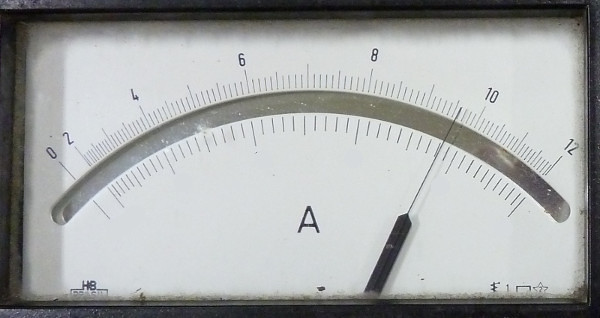The image is of an ammeter, designed as a rainbow-shaped arc with a white face. The ammeter's scale is marked with numbers in increments of two, ranging from 0 to 12. Currently, the needle points precisely at 9.6, indicating the measured current. Prominently displayed on the meter is a capital letter 'A,' suggesting it measures amperage. The black letters, numbers, and division lines contrast sharply with the white background, ensuring clear visibility. A protective plastic cover encases the meter. At the bottom of the ammeter, "HB BRAZIL" is written in capital letters, alongside an electric symbol, the number '1', a rectangle, and a star.